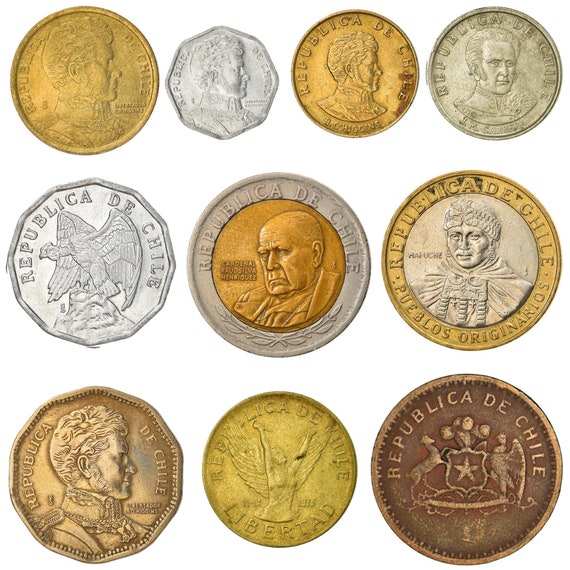This color photograph features a collection of coins in three rows, presumably Chilean currency given the consistent wording "Republica de Chile" on each coin. The coins vary in shape and color, with tones ranging from gold, silver, bronze, to dark brown. Most of the coins are circular, but some have unique shapes, including an octagon and other polygonal forms.

In the top row, there are four coins:
1. A gold coin featuring a man looking to the right.
2. An octagonal silver coin with the same man in the same pose.
3. Another gold coin showing the same man.
4. A silver coin with the same man now looking directly at the viewer.

The second row consists of three coins:
1. A silver coin depicting a large bird perched on a rock.
2. A coin with a silver rim and a bronze center showing a stern-looking bald man, likely Cardinal Faustino Enriquez, looking to the left.
3. A coin illustrating a person in ceremonial dress, labeled "Pueblos Originarios."

The bottom row includes three coins:
1. A coin with a man in military uniform looking to the right.
2. A gold-toned coin showing an angel reaching towards the sky, marked "Libertad."
3. A dark brown coin displaying a deer and an eagle surrounding a shield.

Overall, the coins display a mixture of historical figures and symbolic imagery, and while most are uniform in their circular shape, a few coins stand out due to their distinctive polygonal forms.